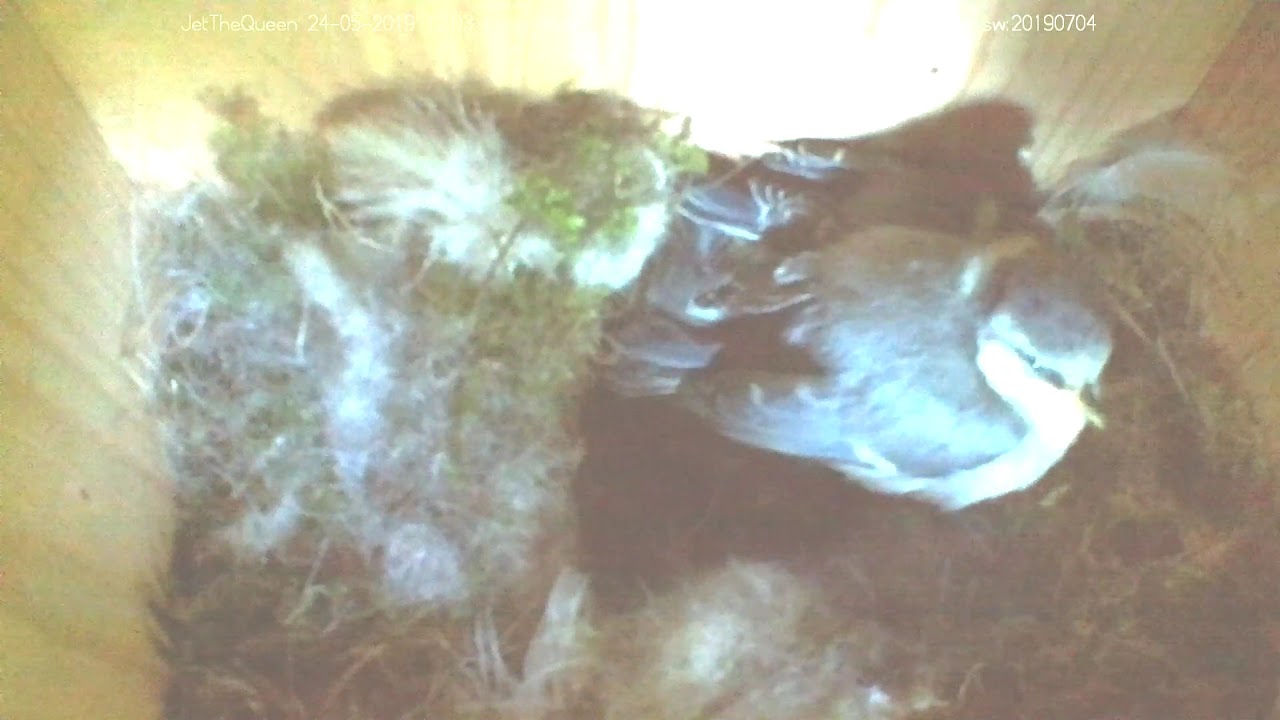This low-resolution, top-down, photorealistic image captures the interior of a bird enclosure with light golden wooden walls. At the top center, there is a brightly lit door to the outside. The floor is covered in dark brown straw-like pieces and dried organic material. Towards the right center, a bird with gray feathers and a white breast, possibly a homing pigeon, is perched. The bird has a dark gray head and slight turquoise shading below it. Behind it, more gray feathers are discernible, though it's unclear if they belong to other birds or are loose feathers. Shadows cast by the bird obscure finer details, such as the possibility of eggs or chicks beneath her. Semi-transparent white text at the top reads "Jet the Queen," along with partially obscured date and location information, "24-05-2019" and "Southwest 201-90-704," capturing a snapshot in time of this serene avian scene.